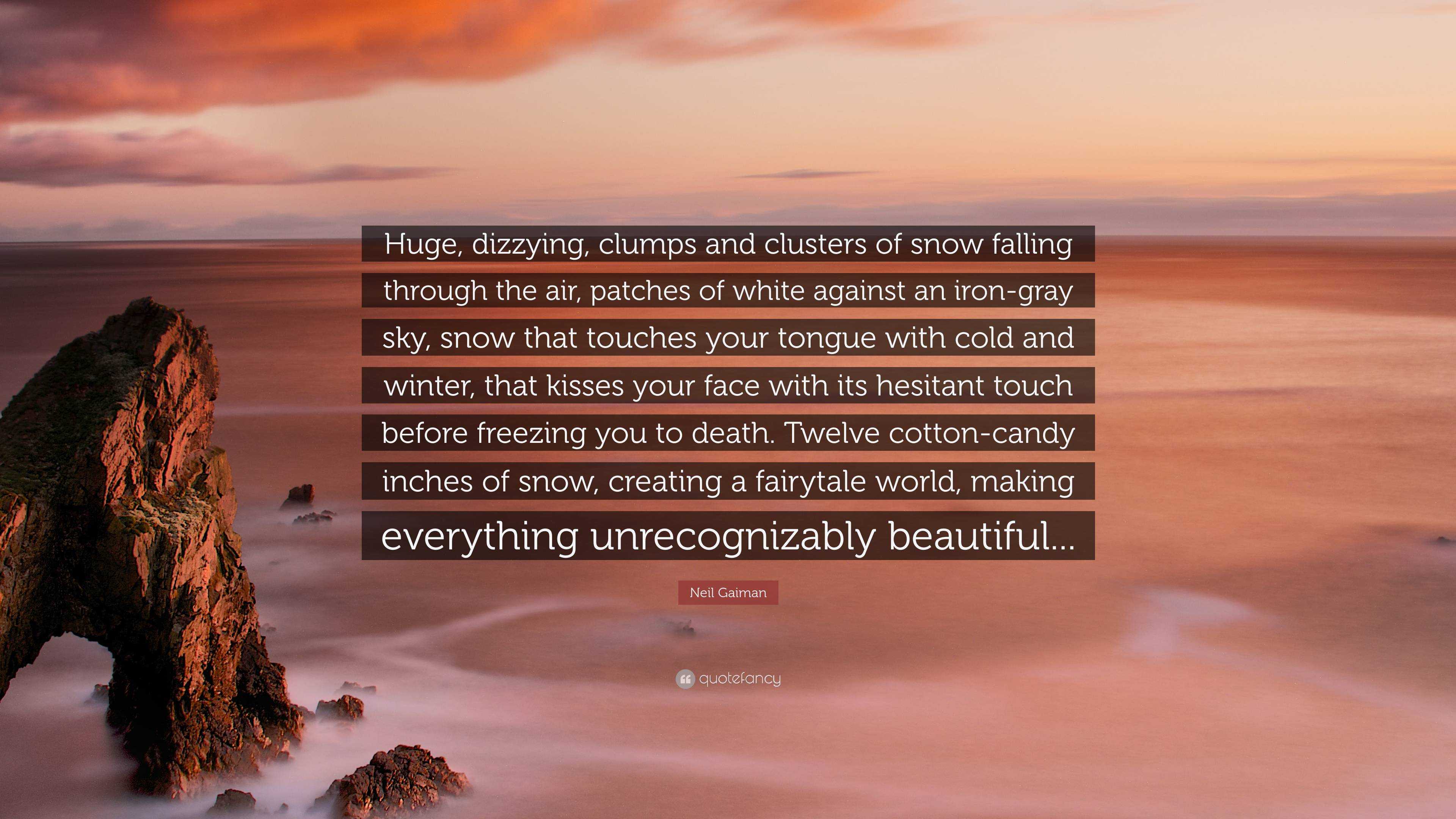The image portrays a surreal outdoor scene steeped in a pink, red, and peach hue with soft light purple and yellow undertones. On the left, there is a notable rock formation that stretches from the bottom left corner up to the midpoint of the image. The sky and clouds share the same pinkish tones, blurring the lines between the different elements. In the center, a series of poetic text lines in white font, each highlighted by a brown backdrop, cascade down the image. The text reads: "Huge dizzying clumps and clusters of snow falling... Through the air, patches of white against an iron gray sky, snow that touches your tongue with cold and winter that kisses your face with a hesitant touch before freezing you to death... 12 cotton candy inches of snow creating a fairytale world making everything unrecognizably beautiful..." Below this poetic imagery, the name Neil Gaiman is inscribed along with the word "quote," within a gray circle marked with white quotation marks, adding a whimsical literary touch to the fantastical scene.